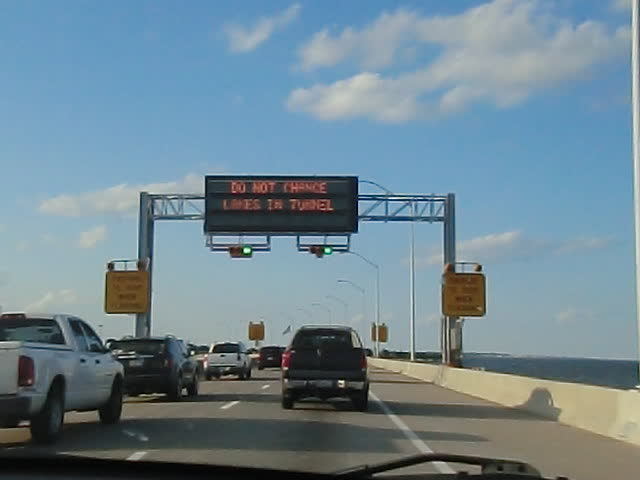This photograph captures the view through a car windshield, looking out onto a stretch of gray asphalt road. The road ahead features a straight white line running down the center, a solid line on the right, and a dotted line on the left, suggesting the approach to a tunnel. A concrete barrier separates the road from a body of dark blue water to the left. Overhead, the sky is a clear blue dotted with fluffy white clouds.

Prominently, a silver metal frame spans across the road, supporting a lit street sign at the top. The sign displays a warning in red text: "DO NOT CHANGE LANES IN TUNNEL." Below the main sign, two yellow caution signs are mounted on either side of the frame, adding to the array of road signage. In front of the vehicle, lines of cars can be seen, indicating moderate traffic on this bridge-like structure. The entire scene suggests a moment of caution and anticipation as drivers prepare to enter a tunnel ahead.